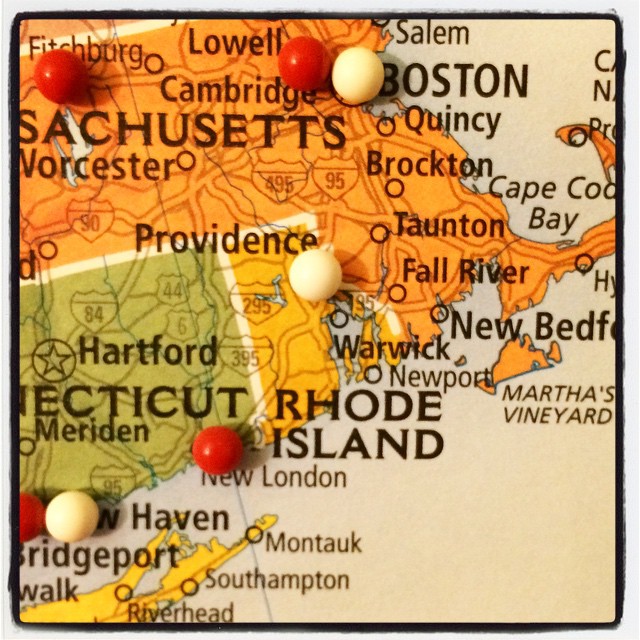This detailed photograph captures a close-up of a pin board map centered on the northeast region of the United States, specifically featuring the states of Massachusetts, Connecticut, and Rhode Island. The entire image has a faded yellow filter around its outer edges, giving the scene a vintage feel. The map is bordered by a light gray outer frame and an inner black border which neatly outlines the states. Massachusetts is presented with black text against an orange backdrop, marked prominently with red and white pushpins in cities such as Fitchburg, Cambridge, and Boston, with that of Boston being white. Below Massachusetts, Rhode Island is highlighted in yellow with a white pushpin in Providence. To the left lies Connecticut, shaded green, showing red pins in New London and Bridgeport, and a white pin in New Haven. Multiple cities such as Newport, Brockton, Salem, and Hartford are also pinpointed. The map intricately details major cities and roads connecting them, with the grayscale indicator to the side representing water. The framing and color differentiation enhance the clarity and emphasis on the specified regions and notable cities connected by major roads.